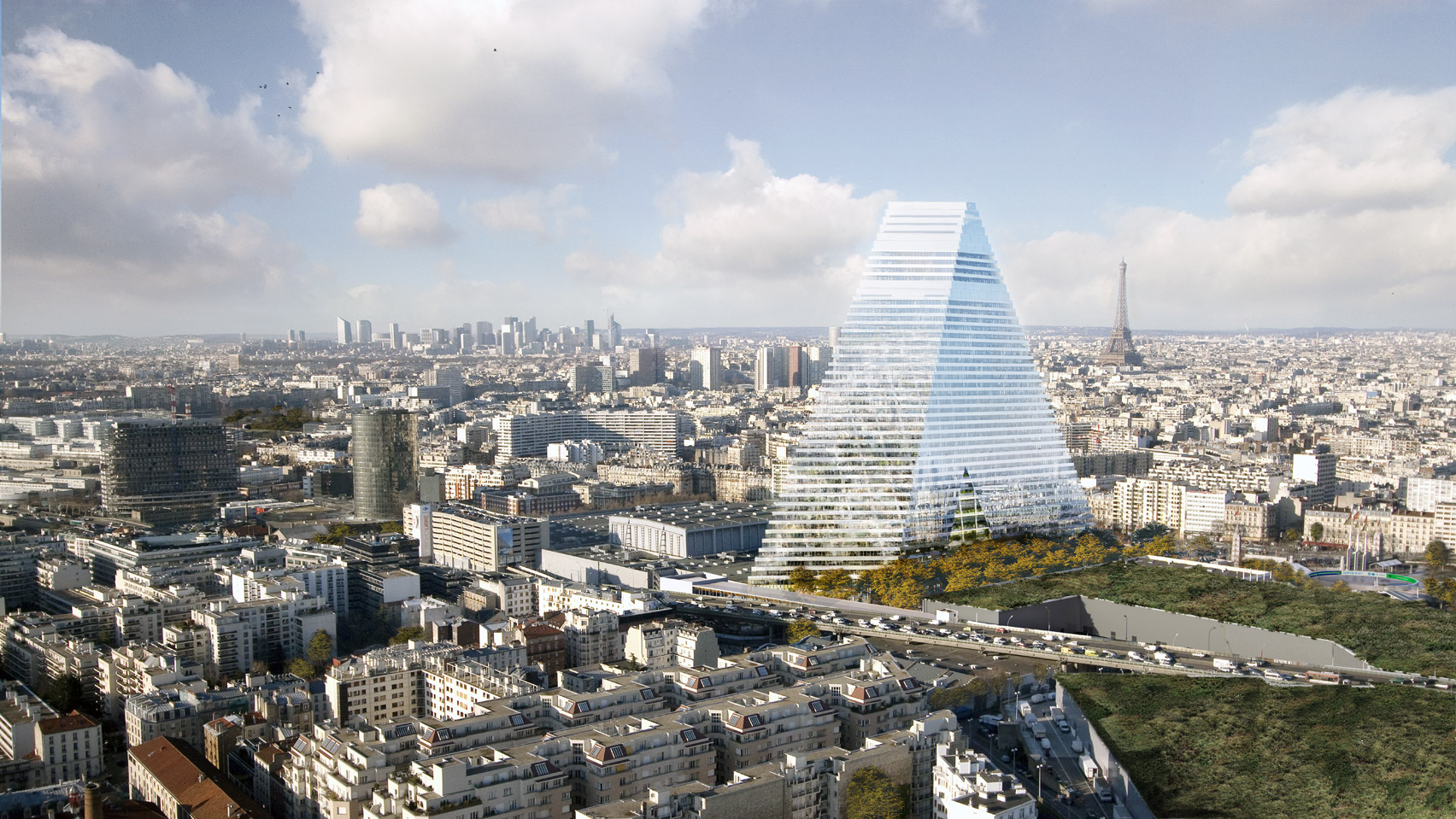The image depicts a bustling cityscape of Paris, captured from an overhead view. Dominating the foreground is a striking, triangular-shaped building with mirrored windows that give it a shiny, reflective appearance. This unusual structure is surrounded by more conventional, densely packed buildings. In the distance, the iconic Eiffel Tower juts confidently into the blue sky, which is dotted with white fluffy clouds. The overall scene is slightly hazy with a grayish tone. Below, a network of roadways, filled with cars, traverses the city, with green shrubbery and grassy hills adding a touch of nature to the urban setting.